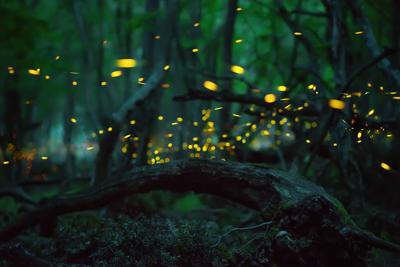In this nighttime forest scene, numerous small glowing orbs – most likely fireflies – create a mesmerizing display with their yellow light, scattered densely throughout the image. These fireflies, slightly blurred due to their movement, form a dazzling contrast against the varying shades of green and gray of the forest under the dark sky. The backdrop features a lush forest with tall tree trunks reaching upward and a lighter green canopy overhead. Dominating the lower portion of the image is a horizontally arched fallen log that stretches across the width of the scene, with green foliage and bushes surrounding it. The fireflies swarm above and between the trees, their glowing dots creating a magical atmosphere amidst the natural landscape.